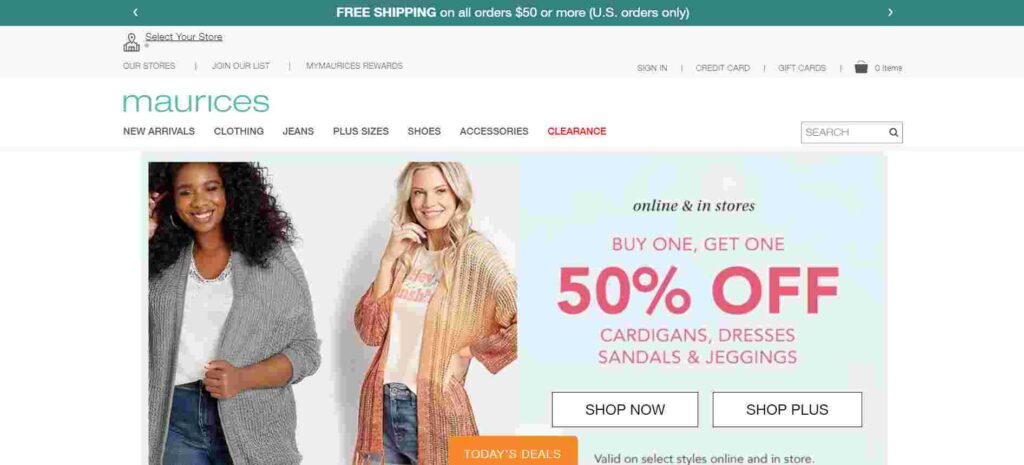This is a descriptive and detailed caption for the image provided:

---

The website from Reese's Designer Clothing department store greets visitors with a prominent promotional banner at the top, offering free shipping on all U.S. orders of $50 or more. This message is displayed in white text against a vibrant green background, forming a green bar across the top. Navigation arrows on either side of the banner suggest more deals can be explored by clicking through.

Directly beneath this banner are various user options, including an option to select a store location, a link to join their mailing list, and sign-in options for members. There's also a section detailing available credit card options and gift cards. The shopping cart icon, presently showing zero items, indicates no products have been added to the cart yet.

The main content of the site begins with the prominent "Maurice's" logo in lowercase teal text. Below this, a bold, black "NEW ARRIVALS" header announces new merchandise categories like clothing, jeans, plus sizes, shoes, accessories, and clearance items, which is highlighted in pink text.

Centrally featured is an image of two women modeling Maurice's apparel. On the right, an African American woman poses thoughtfully, holding her hair and clutching her ribbed, button-up gray sweater layered over a white shirt, paired with jeans. To her left, a blonde Caucasian woman gazes ahead with a hand raised to her face, dressed in a stylish top. 

Text beside the models promotes a "Buy One Get One 50% Off" sale applicable to items like cardigans, dresses, sandals, and leggings or jeggings. This message is accentuated with large, bold typography. Below this offer are functional buttons for 'Shop Now' and 'Shop Plus.'

An orange button placed over the blonde model reads "Today's Deals" in white text, and a note underneath clarifies that the deals are valid on select styles both online and in stores.

---